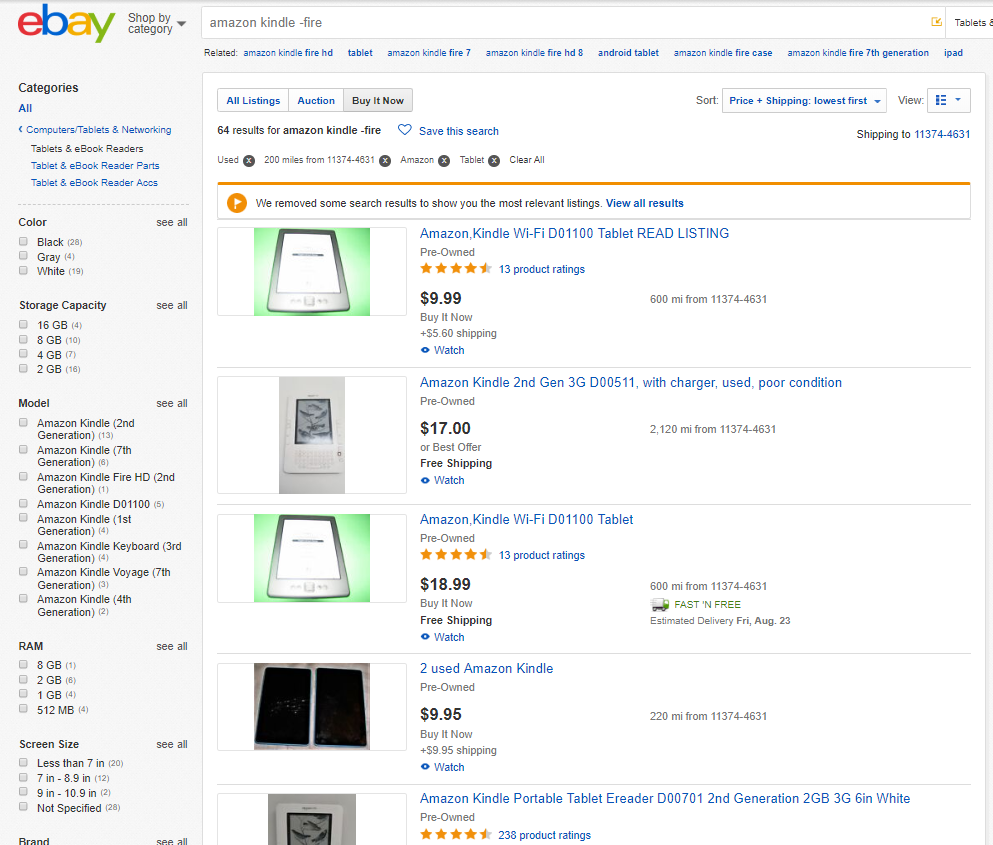The webpage displays eBay's website, focused on the search results for "Amazon Kindle Fire." The results are filtered under the "Buy It Now" option. Prominently, an orange circle contains a flag icon, next to which a note explains that some search results were removed to show the most relevant listings, with an option in blue text to “View all results.” The listings displayed include several Amazon Kindle devices: the first priced at $9.99, the second at $17, the third at $18.99, and the fourth at $9.95. Below the search bar, additional related searches are shown in blue text, including "Amazon Kindle Fire HD tablet," "Amazon Kindle Fire 7," "Amazon Kindle Fire HD 8," "Android tablet," "Amazon Kindle Fire case," and "Amazon Kindle Fire 7th generation." The shipping destination is indicated as 11374.